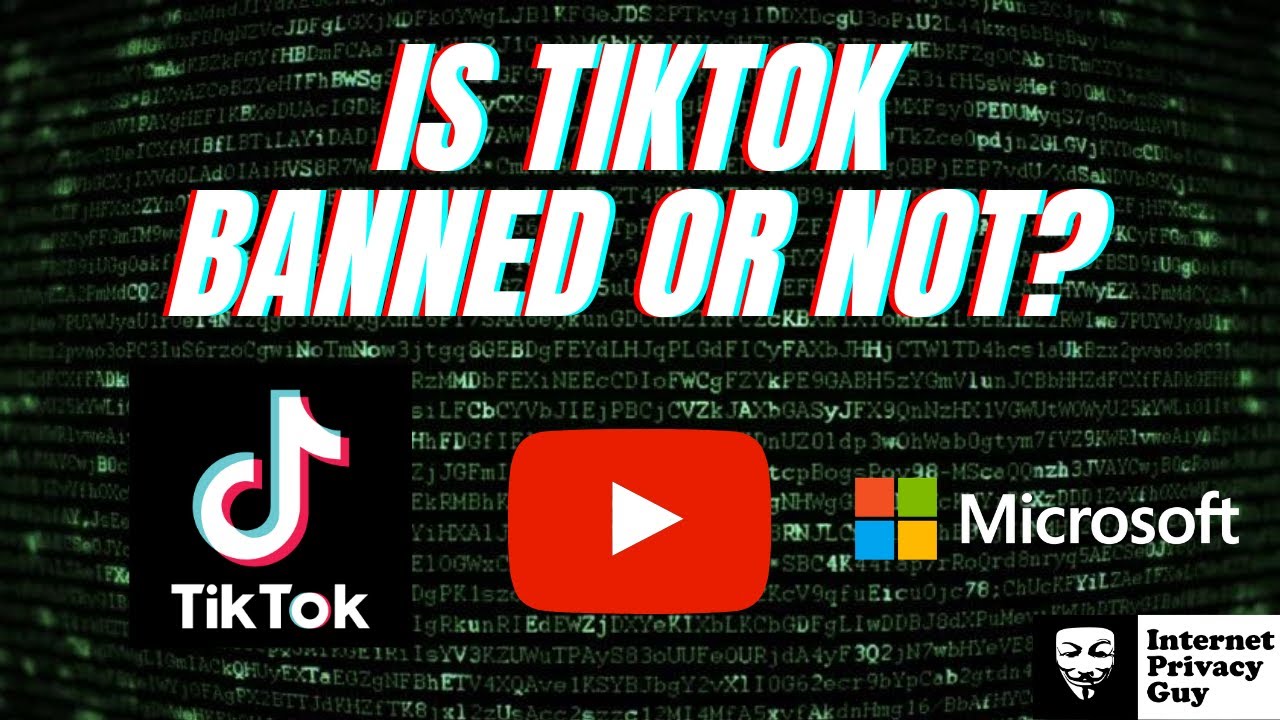This image resembles a TikTok-themed visual, featuring a bold question on the topic of platform bans. The background is adorned with green, matrix-like lines of letters flowing horizontally, with each line slightly bending and blurring at the ends, accentuating a digital, computer-binary aesthetic. Dominating the upper center of the image, large, white uppercase text reads "TIKTOK." Just below, the question "BANNED OR NOT?" is prominently displayed in the same font style. The lower section of the image showcases three notable logos: starting from the left is the TikTok logo within a black square, followed by the iconic red and white play button of YouTube, and lastly, the colorful windowpane logo representing Microsoft.